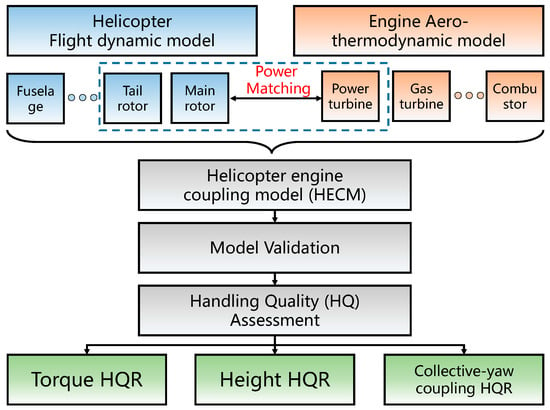This detailed, descriptive caption combines elements from the given input for a comprehensive summary:

The image is a flowchart diagram detailing the Helicopter Flight Dynamic Model and Engine Aerothermodynamic Model. It begins with two equally-sized rectangles at the top, one with a blue background labeled "Helicopter Flight Dynamic Model" and one with an orange background labeled "Engine Aerothermodynamic Model." Below the blue rectangle are three smaller blue squares labeled "Fuselage," "Tail Rotor," and "Main Rotor," and below the orange rectangle are three smaller orange squares labeled "Combustor," "Gas Turbine," and "Power Turbine." A double-headed black arrow with the red text "Power Matching" connects the "Main Rotor" and "Power Turbine." A dotted blue rectangle encompasses the "Tail Rotor," "Main Rotor," and "Power Turbine" boxes, with dotted lines linking "Fuselage" to "Tail Rotor" and "Gas Turbine" to "Combustor." All these elements feed into a gray box labeled "Helicopter Engine Coupling Model (HECM)" via a horizontal bracket. Below this, a sequence continues with a small arrow leading to another gray box labeled "Model Validation," and a subsequent arrow points down to a third gray box labeled "Handling Quality (HQ) Assessment." From here, a three-headed arrow directs to three green rectangular boxes aligned horizontally, each labeled "Torque HQR," "Height HQR," and "Collective Yaw Coupling HQR." This diagram visually represents the interaction and flow between various dynamic components and their roles in helicopter model validation and handling quality assessment.